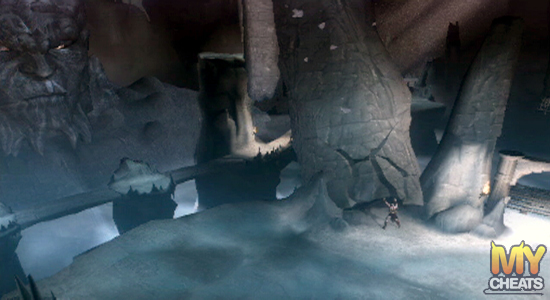The digitally drawn image, presented in landscape orientation, depicts an underwater scene rendered in muted gray and brown tones. Resembling a TV screen from a video game, the bottom right corner prominently features "M-Y" in oversized yellow-orange letters, beneath which "cheats" is written in white.

The scene captures a cavernous underwater environment filled with large, submerged rocks. On the stone ground in the background to the left, a colossal stone face gazes outward. This face, located in the upper left, resembles a man's with its distinct gold eyes, pronounced nose, closed mouth, and detailed depiction of a beard and long hair.

In the foreground, slightly right of center, stand three substantial stone pillars—one at the center and two flanking it. Dominating the space in front of the largest pillar is a diminutive figure of a man. Bare-chested and clad in a skirt and boots, he raises his arms as though lifting the boulder or pillar before him, adding an element of dynamic effort to the enigmatic, submerged setting.